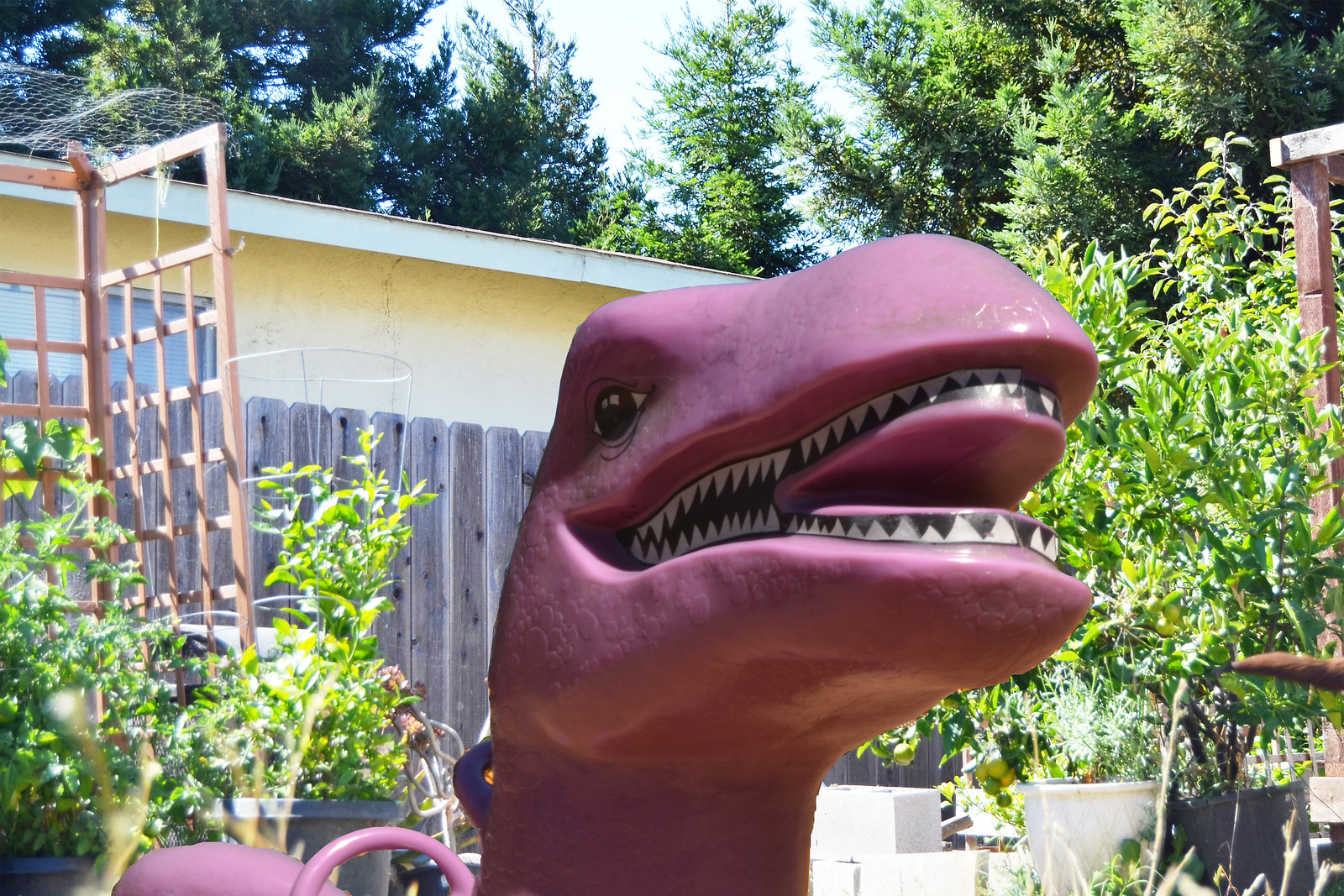The photo captures a whimsical scene set outdoors, possibly in a park or backyard, featuring a standout artificial dinosaur statue. The statue, likely made of plastic or a similar material, is primarily a deep dark purple color with distinct black and white detailing in its open mouth. Sharp, triangular white teeth and a dark black eye contribute to its playful, novelty appearance. The dinosaur's open mouth reveals a black interior, adding a touch of charm to its exaggerated features. Surrounding the statue, tall, verdant trees and a variety of potted plants create a lush backdrop. A small wooden trellis for climbing plants is positioned to the left, enhancing the garden-like ambiance. In the bottom left corner, a hint of a pink object—possibly a water bottle or a flamingo decoration—adds a splash of color and curiosity to the image.